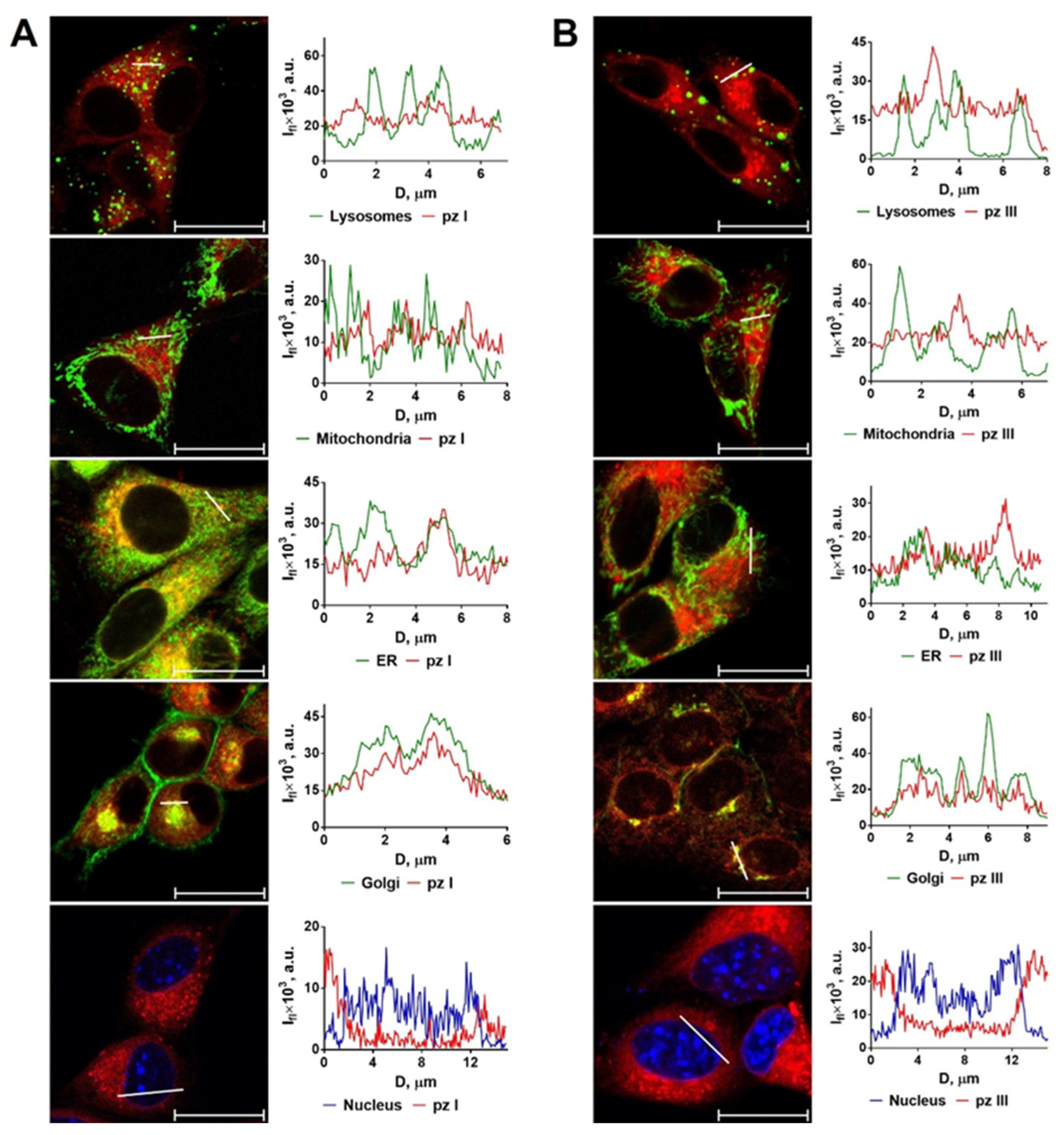The image presents a detailed series of scientific scans that look like they belong in a research paper. There are two columns labeled A and B, each containing five microscopic images and accompanying graphs. The images, which appear to be cellular in nature, are arranged vertically within each column. 

In Column A, the five images showcase dark backgrounds with brightly colored cells and structures highlighted in shades ranging from yellow to red, green, and blue. To the right of each cell image in Column A is a corresponding graph with squiggly lines, measuring various cellular components. These graphs are labeled with terms such as lysosomes, mitochondria, Golgi, nucleus, and more, and have axes labeled from 0 to 6 horizontally and 0 to 60 vertically.

Column B mirrors Column A in format, with another set of five cellular images and corresponding graphs. The graphs in Column B also display colored lines and have similar labels to those in Column A, indicating a consistent set of measurements or comparisons across the two columns.

Each image in both columns is detailed with cellular structures, and the graphs beside them provide a visual representation of data concerning these structures. Overall, the images and graphs are colorized and intricately labeled, giving off a highly specialized, scientific feel.